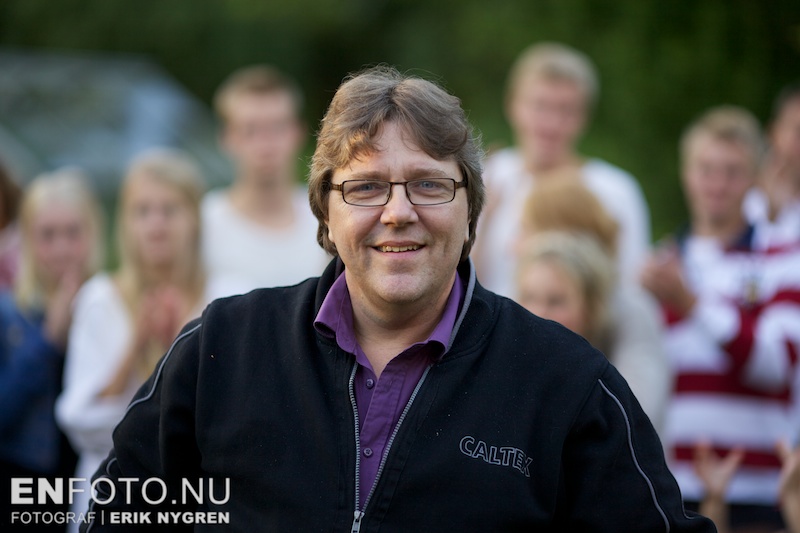This outdoor image captures a close-up of a smiling man wearing brown, rectangular-framed glasses and a blue jacket that appears to read "CALTEX" or "CALTECH." The jacket is partially unzipped, revealing a purple button-up shirt with the top two buttons undone. The man's hairstyle is reminiscent of the 1970s or early 1980s, with swept bangs on both sides of his face.

In the blurred background, there is lush green foliage and a possible building. The out-of-focus group consists of at least seven people, mostly dressed in white shirts. Among them, one individual is wearing a white shirt with red stripes, and another appears to be sporting a blue sweater. The group seems to be applauding, with their hands positioned as if clapping. 

In the bottom left corner, there is a watermark that reads "Enfoto.nu" and "Fotograf Erik Nygren."